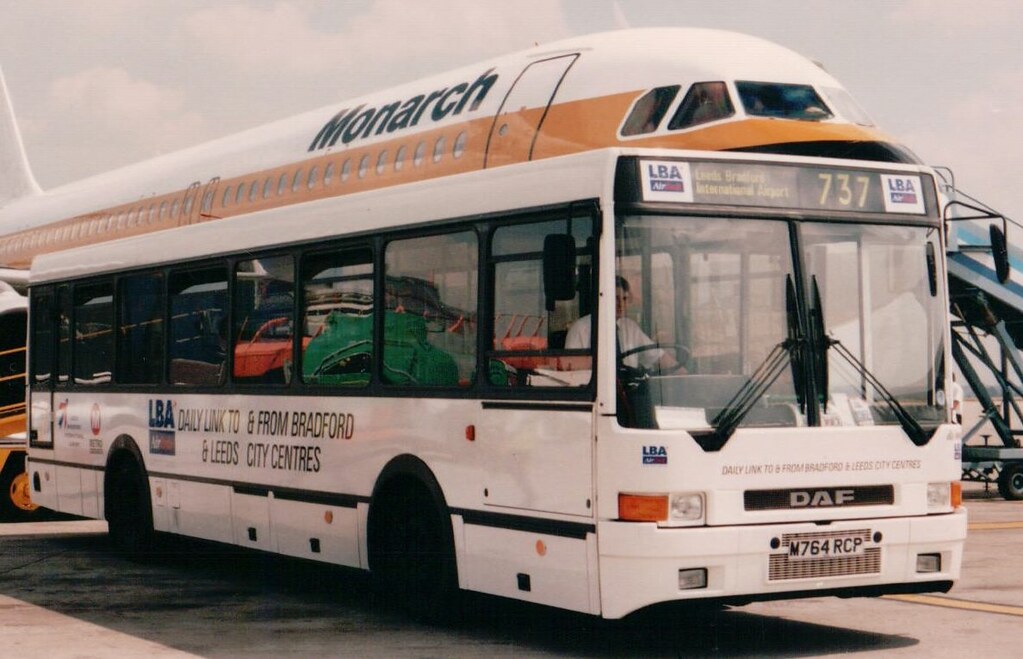A vintage photograph showcasing an aged, slightly brown-tinted texture captures an aviation scene at an airport. Dominating the foreground is a white, blocky shuttle bus with black tires and the label "DAF" on the front, while the side advertises, "Daily Link to and from Bradford and Leeds City Centers." The bus, identified as route '737,' is stationed on the tarmac, indicating it services passengers from nearby hotels or various destinations. Behind and just above the bus, an orange and white Monarch passenger jet, marked with a prominent orange stripe and black "Monarch" lettering, is parked and appears to be in the process of boarding or deboarding through a visible ramp. The driver of the bus, dressed in a white short-sleeved button-down shirt and black tie, is seen behind the wheel, ready to transport passengers either to or from the aircraft situated at Leeds-Bradford International Airport.